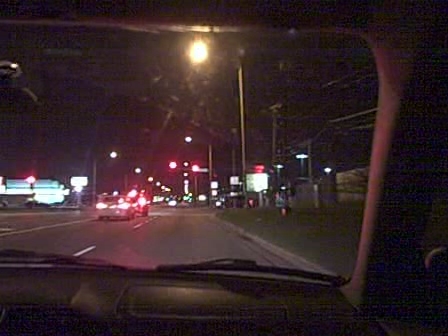From the perspective of a passenger in the front seat, this nighttime photo captures a roadway extending into the distance, lit by numerous streetlights that line both sides. The black dashboard is seen at the bottom, adding context to the inside view of the vehicle, which features a reddish-brownish interior. Windshield wipers are faintly visible in the background, indicating the passenger side. 

Up ahead, there's an intersection with two illuminated red traffic lights, where a couple of cars in the left lane have stopped, their brake lights brightly visible. White dotted lines delineate the lanes. The view also includes several lit-up store signs and buildings, primarily on the left and right sides of the road, with a conspicuous large white sign topped by a red one on the right. Telephone poles and possible electrical wires are faintly outlined in the background, contributing to the urban night scene.